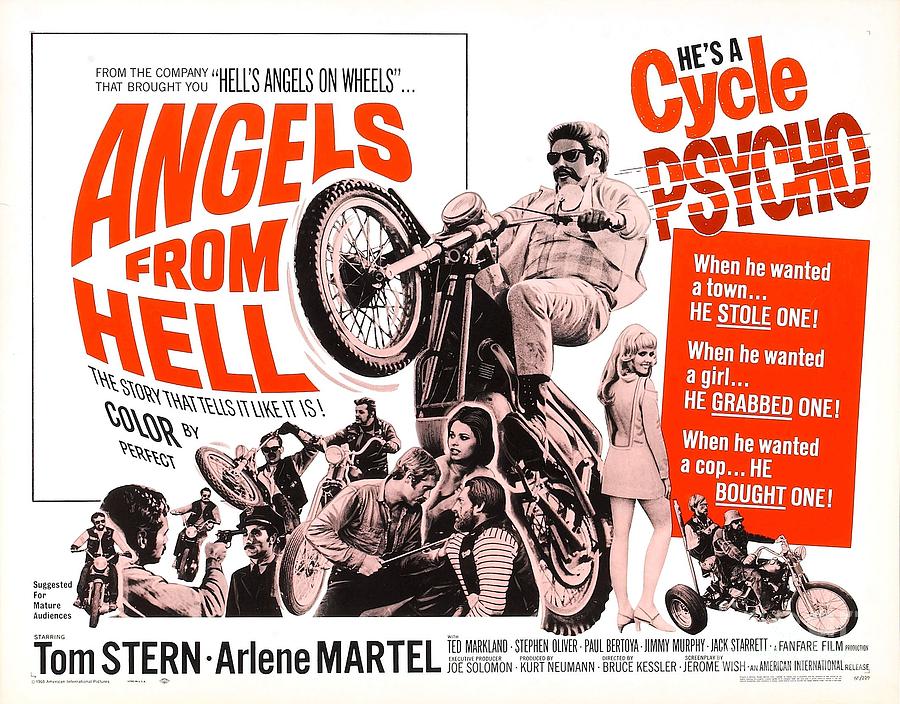The image is a detailed poster for the movie "Angels from Hell." Dominating the scene is a man on a partially lifted motorcycle, donning sunglasses, a mustache, a flannel shirt, a jacket, pants, and boots. In the upper left corner, text on a white background proclaims, "From the company that brought you Hell's Angels on Wheels." The movie title, "Angels from Hell," appears prominently in large red lettering. Below this, in black lettering, it states, "The story that tells it like it is," followed by "Color by Perfect."

To the right, bold text declares, "He's a Cycle Psycho." An orange or reddish rectangle follows with white lettering detailing, "When he wanted a town, he stole one. When he wanted a girl, he grabbed one. When he wanted a cop, he bought one." Images around the central figure include men riding motorcycles and a woman in a short dress and high-heeled shoes, looking over her shoulder. At the bottom, in black lettering, are the names of the stars, Tom Stern and Arlene Martel, along with a note suggesting the movie is "suggested for mature audiences."